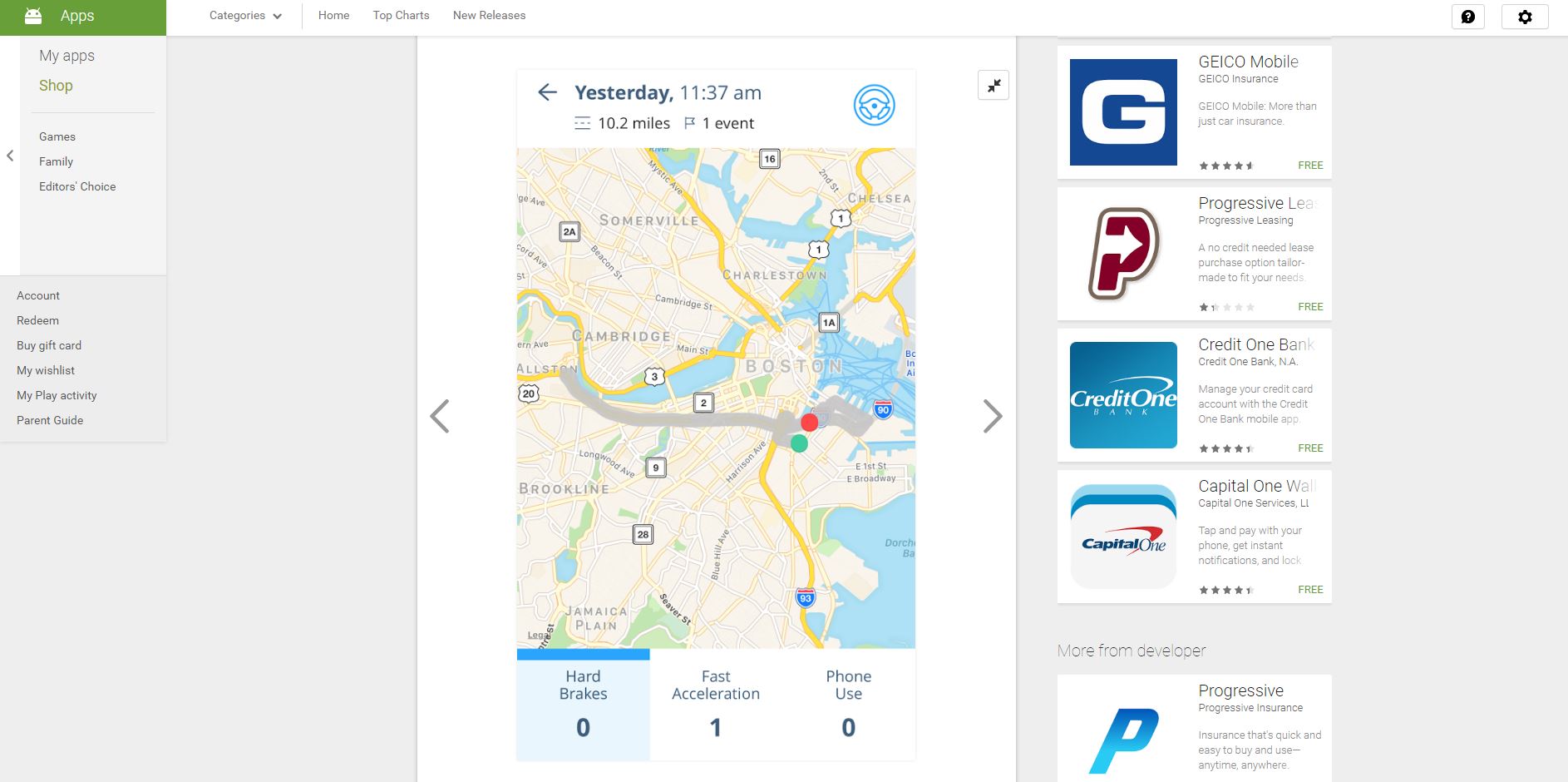The image shows a user interface with several key elements:

**Top Section:**
- A green button labeled "Apps" is prominently featured at the upper part of the interface.
- A drop-down menu under this button contains options such as "My Apps," "Shop," and possibly "Family," although the text is blurry and somewhat hard to read.

**Middle Section:**
- On the right side, there is a map with a white outline displaying a certain location near a bay area that is intersected by multiple interstate highways.
- An informational text snippet reads: "Yesterday, 11:37 AM, 10.2 miles, one event."
- Below this, there are performance metrics: "Hard brake: 0," "Fast acceleration: 1," and "Phone use: 0."

**Bottom Section:**
- Information boxes are listed in descending order:
  - "Geico Mobile" with the company's logo and information.
  - Another box labeled "Progressive."
  - Followed by boxes for "Credit One Bank" and "Capital One Bank."
- There is a link labeled "More," with an additional line that reads "More from developer: Progressive."

The interface appears to focus on app management combined with real-time tracking data and promotional content from various financial and insurance companies.